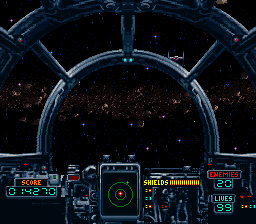A mesmerizing scene from a video game showcases a meticulously designed spaceship cockpit, adorned with intricate graphics and stunning details. At the forefront, a circular main window draws the viewer's gaze, framed by four rounded rectangles and an additional outer layer. Through this window, the expanse of space unfolds, revealing a distant spaceship amidst a breathtaking star-studded backdrop. Dominating the center of the view is a vibrant Milky Way-like formation, characterized by red-hued rocks and a contrasting field of white stars surrounding it.

The cockpit’s dashboard is particularly striking, featuring a central device reminiscent of an iPad. This screen displays a targeting interface with a prominent red bullseye, alongside crucial in-game metrics: a score of 14,270, 20 enemies, and 99 lives remaining. A fully charged shield indicator reassures the player of their defenses. Below the screen, the flight navigation stick is subtly visible, underscoring the interactive nature of the game and immersing the player in their intergalactic voyage.